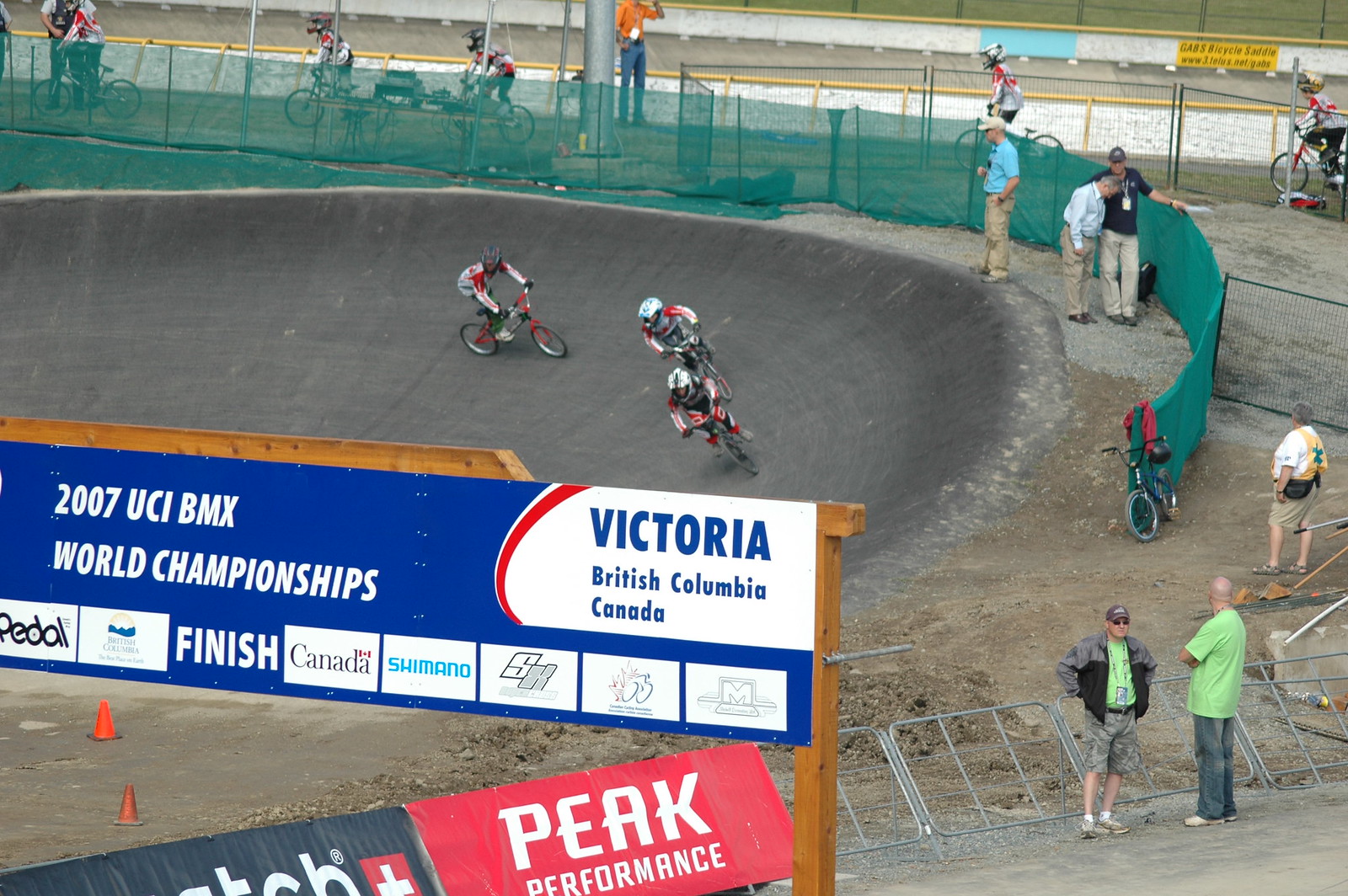The image captures a top-down view of the 2007 UCI BMX World Championships held in Victoria, British Columbia, Canada. The focal point is a gray asphalt racetrack which features a steep incline, curving inwards with the outer edge significantly elevated. Three cyclists are visible on the track, all riding red and black bikes and wearing coordinated outfits of white, red, and black. In the distance, more cyclists dressed in similar red and white long-sleeve shirts with black helmets can be seen. The track area is surrounded by a green chicken wire fence supported on black poles, accompanied by sections of silver metal fencing. Various people, both with and without bicycles, are standing around the track, which also features sponsorship signage, including "Shimano Canada". Cones are scattered around, and the event branding "2007 UCI BMX World Championships, Victoria, British Columbia, Canada" is prominently displayed in the foreground. The scene is bustling with activity and anticipation as the race unfolds.